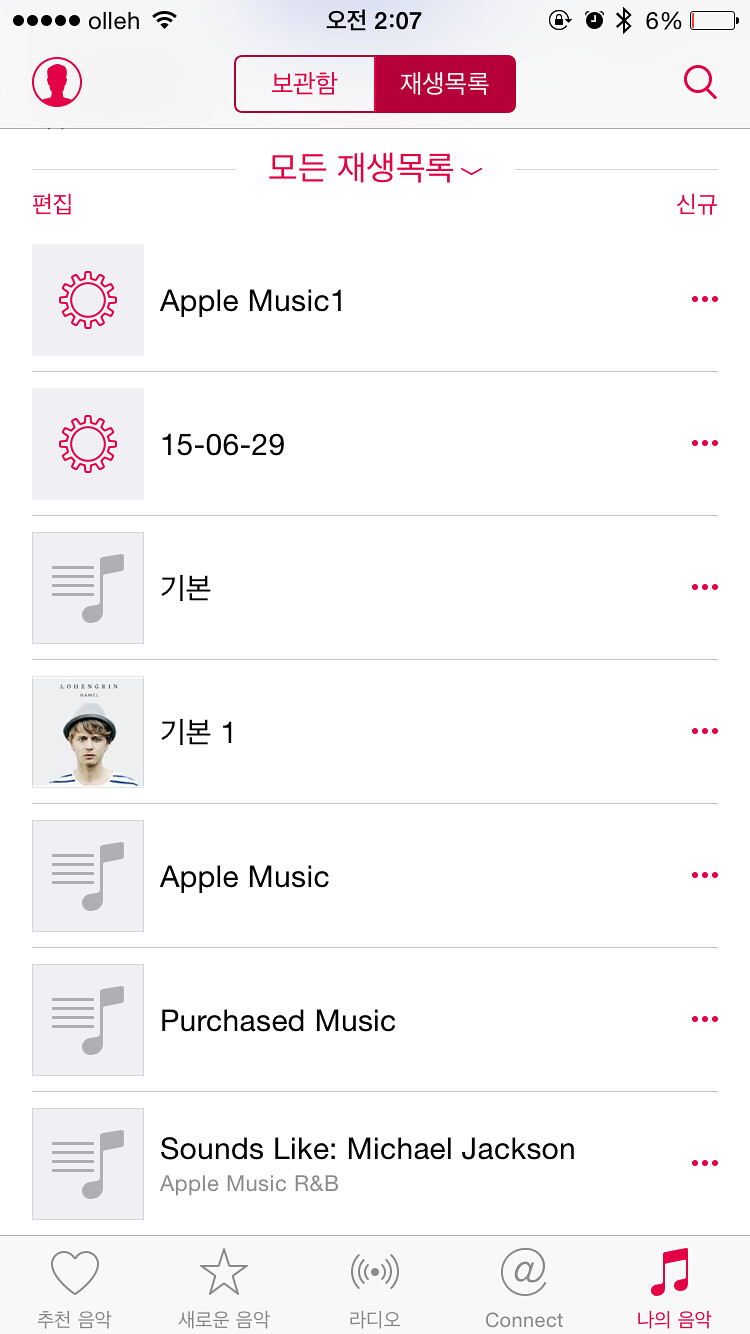The image shows a screenshot of an iPhone displaying the Apple Music app in what appears to be an Asian language. The interface has a light gray banner at the top indicating a time of 2:07, a low battery level of 6%, and various icons such as Bluetooth and Wi-Fi, with the Wi-Fi labeled as O-L-L-E-H. Below the banner is a half-white, half-magenta border with Asian characters—white text on magenta and magenta text on white. The main content includes a white background with more Asian lettering and various icons and labels. These labels include English text examples like "Apple Music 1", "15-06-29", "Purchased Music", and "Sounds Like Michael Jackson," indicating Apple Music Rhythm in Blue genre. Towards the bottom, there's a horizontal banner featuring icons such as a heart, star, speaker, @ symbol, and a highlighted magenta musical note with additional text. Each row in the list seems to correspond to different music categories or playlists, blending between languages.